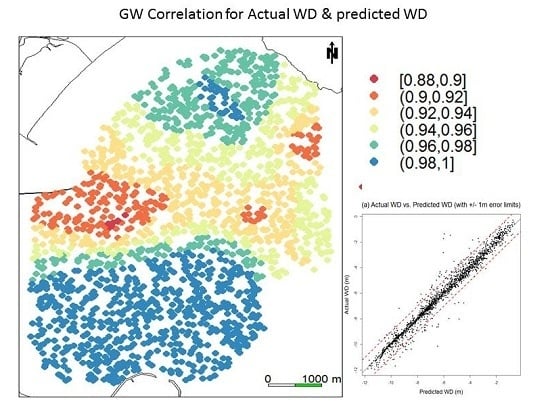This image features an intricate educational graph titled "GW Correlation for Actual WD and Predicted WD." At the center-left of the image, there's a prominent scatter plot composed of circles or squares in various colors, including blue, green, light green, dark yellow, orange, and red. Below this scatter plot, a horizontal axis spans from 0 to 1,000 meters (M), while a vertical axis runs alongside with an N pointing upwards, indicating north.

On the right-hand side of the image, an indicator or legend lists the colors with corresponding numeric values: red (0.88 to 0.90), orange (0.90 to 0.92), dark yellow (0.92 to 0.94), light green yellow (0.94 to 0.96), green (0.96 to 0.98), and blue (0.98 to 1), illustrating the correlation between colors and specific ranges.

In the bottom-right corner, there’s another graph with black dots arranged diagonally, labeled "Actual WD vs Predicted WD with ±1 M Error." The x-axis is marked as "Predicted WD," while the y-axis is designated "Actual WD." This inset graph highlights the relationship between the actual and predicted water depths, showcasing the accuracy and potential error margin of the predictions.